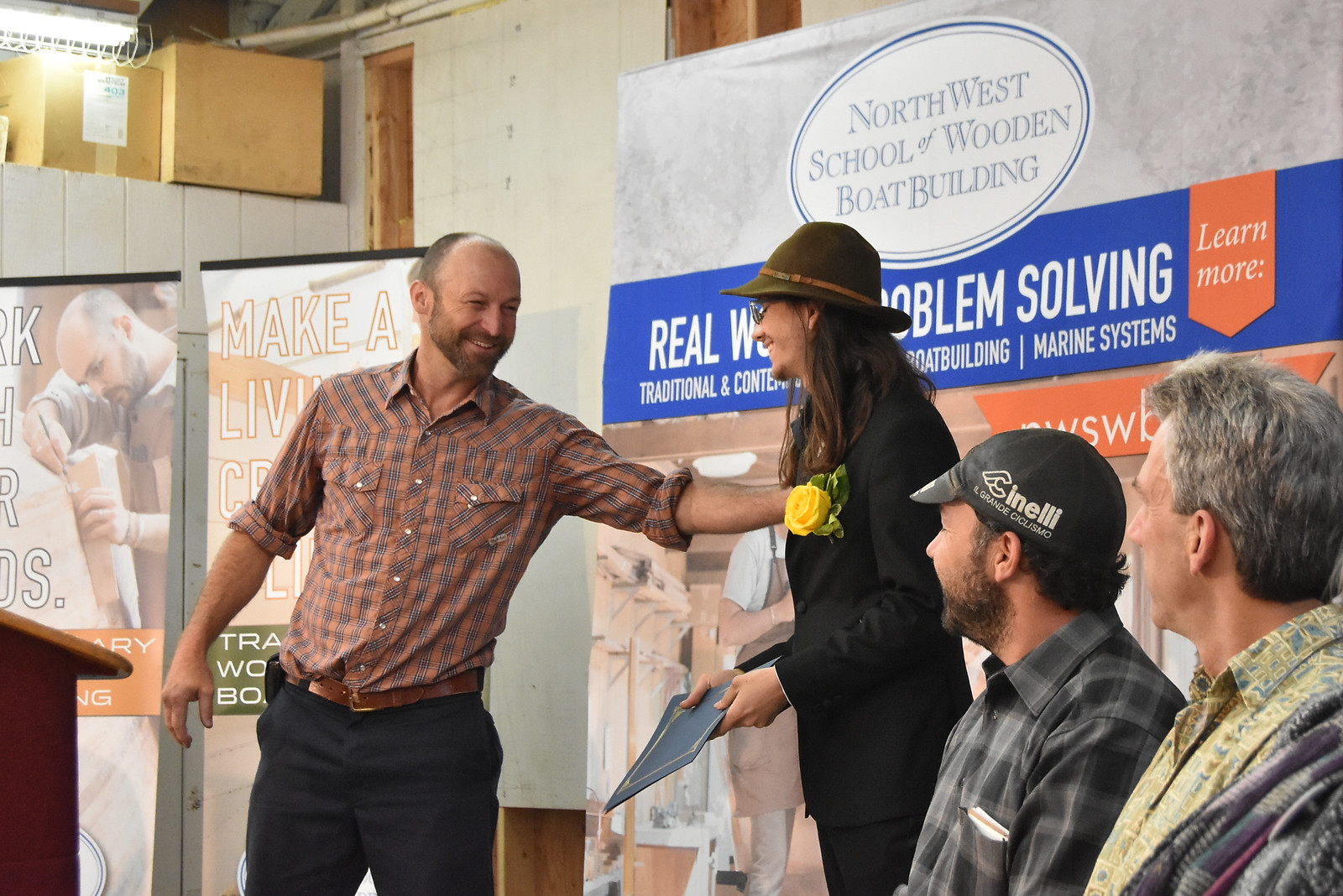This photograph captures a celebratory moment at an event for the Northwest School of Wooden Boat Building. Central to the image is a graduate, a man with long hair, glasses, and a goatee, wearing a black suit adorned with a beautiful yellow rose and green leaves. He also has on a green hat. The graduate, holding his certificate, is being congratulated by another man who has a bald head, a beard, and is wearing an orange and black checkered plaid shirt with black pants. This man is smiling warmly as he reaches out to touch the graduate on the shoulder.

In the background, there is a large banner with text in blue and white that reads: "Make a Living," "Northwest School of Wooden Boat Building," "Real World Problem Solving," "Traditional and Contemporary Boat Building," and "Marine Systems." This banner serves as a backdrop, indicating the educational and celebratory nature of the event.

To the right, sitting down and looking on with smiles are two other men. One man wears a black, white, and gray plaid shirt and a hat labeled "Enel." The other man has salt-and-pepper hair and is dressed in a yellow and blue collared shirt with a jacket. The photograph exudes an atmosphere of achievement and joy with everyone's expressions reflecting the moment's significance.